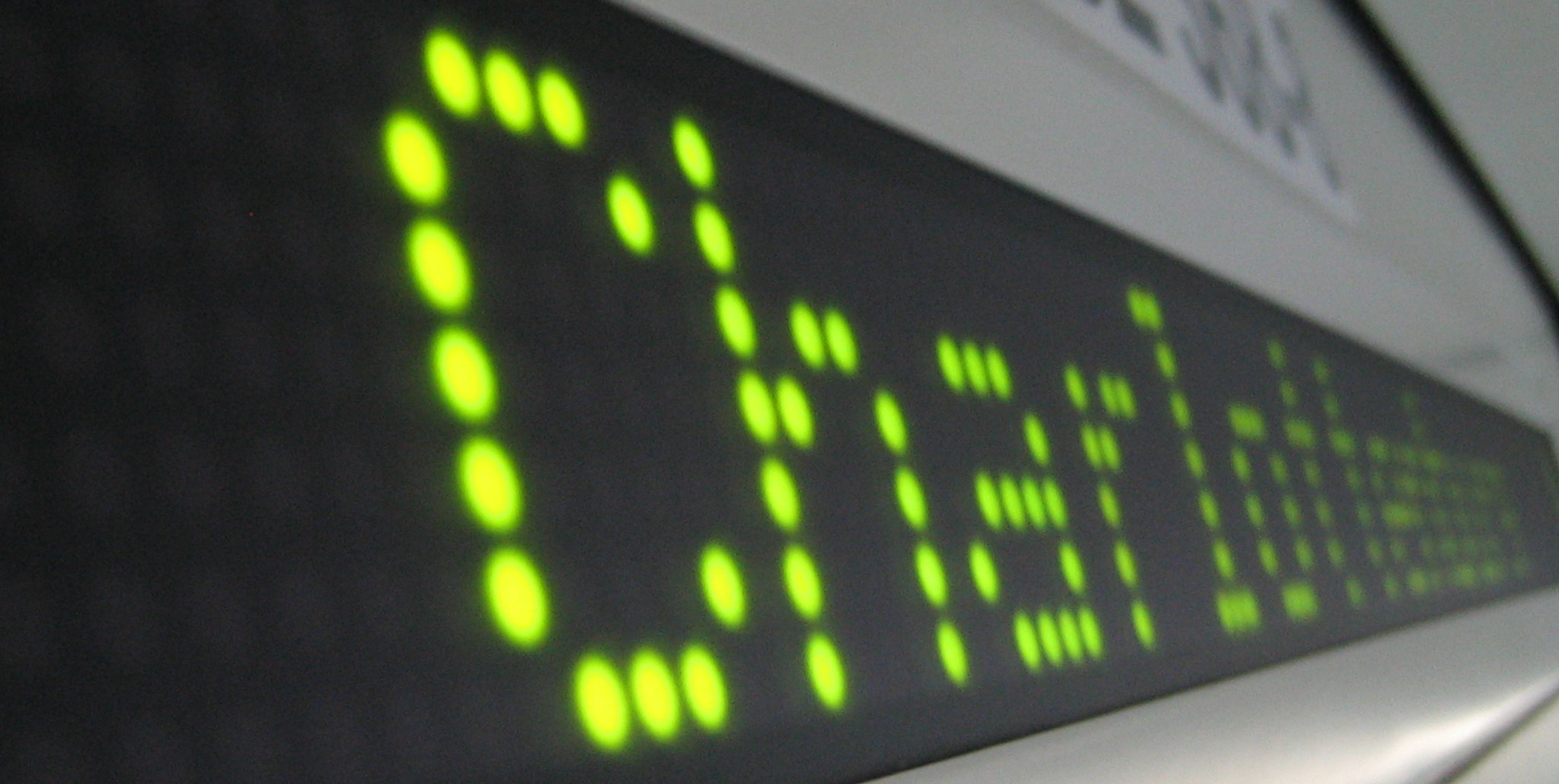The photograph captures an up-close view of an LED sign inside a train station or bus depot, with a focus on the intricate details. The sign displays text made up of bright green dots, likely indicating a destination starting with "CHARL," possibly "Charlton" or "Charlatan." Positioned at an angle, the black background of the LED sign contrasts with the bright green lettering. Embedded into a plain, gray interior with a satin sheen, the sign is placed below a blurry sticker or label, suggesting additional information like a car or bus number. Light filters in from the bottom right corner, illuminating the scene and highlighting the functional, yet unadorned interior design.